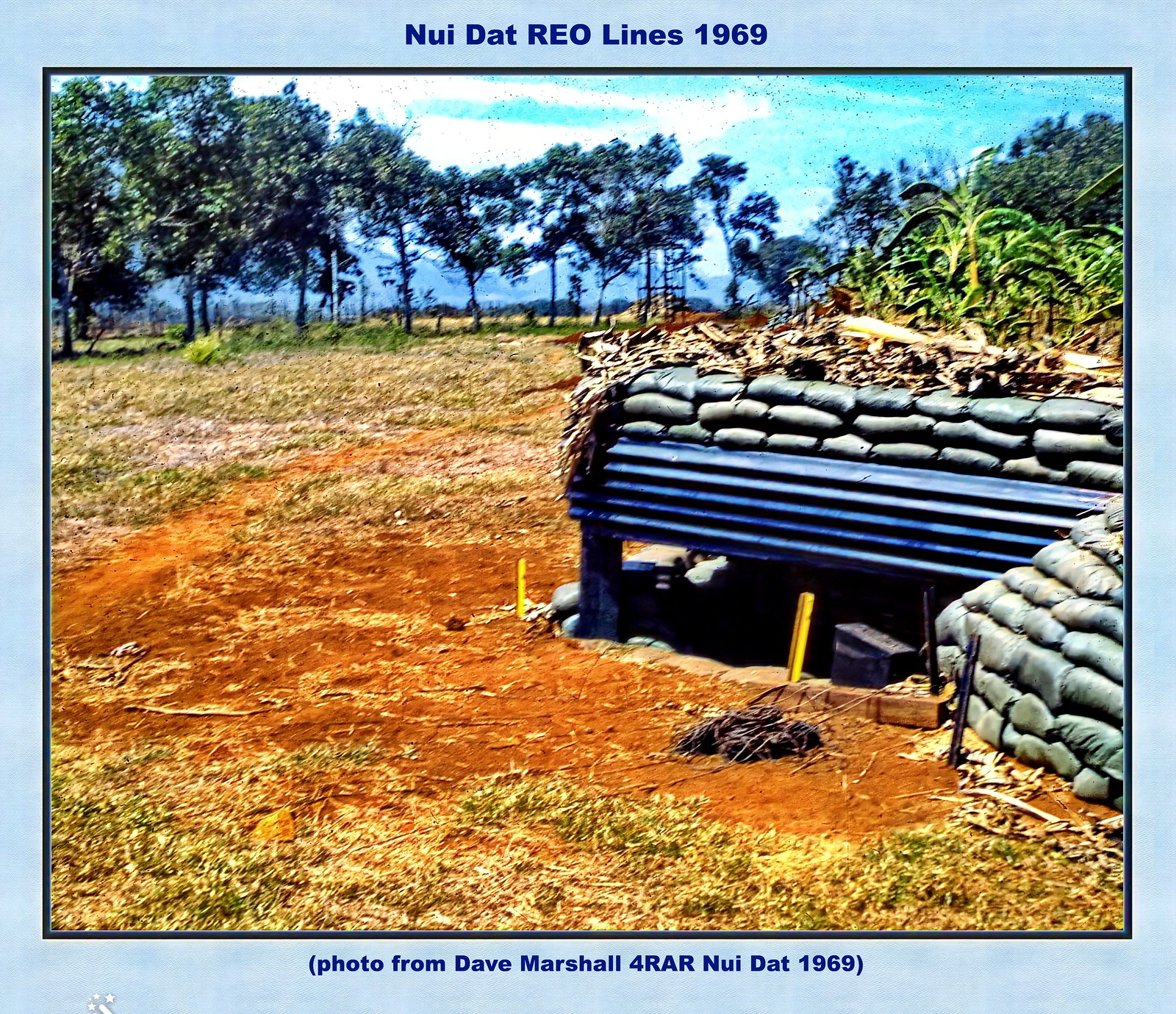This image is a digital photograph of a military bunker situated in an outdoor ground area. On the left side of the photograph, the ground is covered with patches of green and dry grass interspersed with brown soil. The right side of the image features a bunker-like structure with metallic, blue-colored walls and sandbags stacked atop its roof. The bunker has an open window at its base. The background includes rows of trees, some scattered plants, and possibly a fence, all under a blue sky adorned with white clouds. The photograph itself has a light blue border, with the text "Noidet, Rio, Lines, 1969" at the top, and "photo from Dave Marshall for RAR" at the bottom. This older picture captures a scene reminiscent of a military base, though no people are present in the image. The predominant colors are blue, dark green, light green, brown, white, and gray.